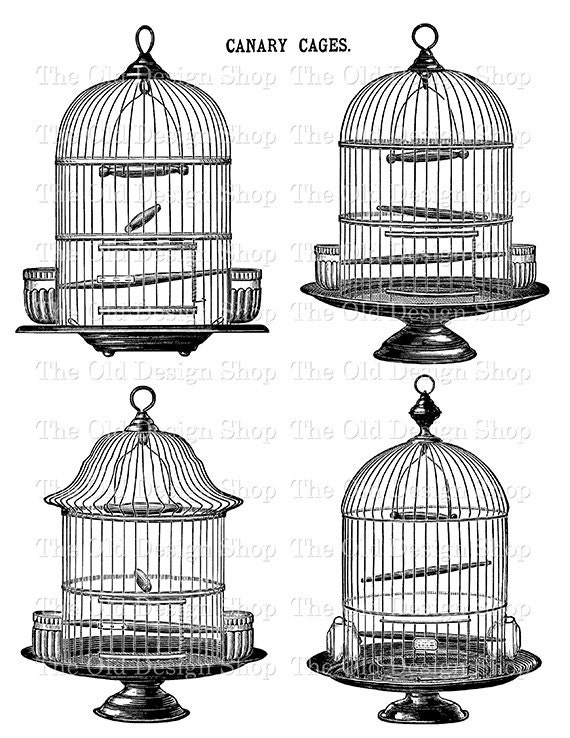The black and white illustration features four distinct canary cages, with the title "Canary Cages" prominently displayed at the top. All four cages embody traditional, classic birdcage designs. The upper left cage has a rounded, dome-like top, small feet at the base, a loop at the top, and an interior swing with some branches. The upper right cage mirrors this design but is elevated on a pedestal instead of having feet. The cage on the bottom left deviates with a pagoda-shaped top and a pedestal base. The bottom right cage returns to the dome shape and also rests on a larger pedestal base. The entirety of the image is rendered in black and white, with no birds or other objects inside the cages. A subtle, light gray watermark reading "The Old Design Shop" spans the background, unobtrusively signifying the source of the illustration.